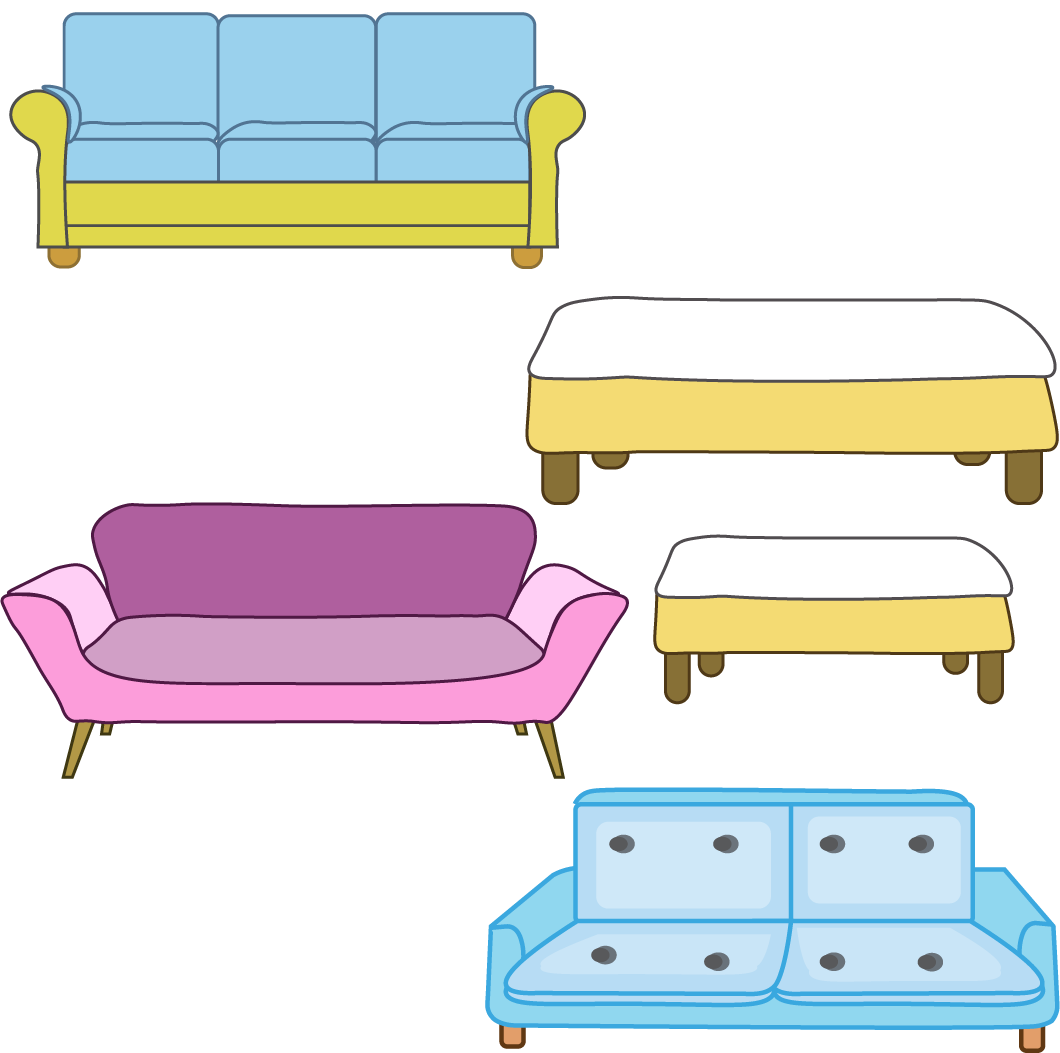The image showcases a collection of computer-generated furniture pieces set against a plain white background. In the upper left corner, there's a sofa with a green base and three blue cushions, each with a click-like design. Directly below it is a modern purple sofa featuring swooping armrests and uniform pink and purple hues, finished with four wooden legs. The bottom right corner hosts a contemporary blue couch adorned with two black dots per cushion, totaling eight, and supported by tan wooden legs. Above this dotted sofa, you'll find two ottomans - the top one being longer and the bottom one shorter. Both ottomans have a white top, yellow sides, and brown legs.